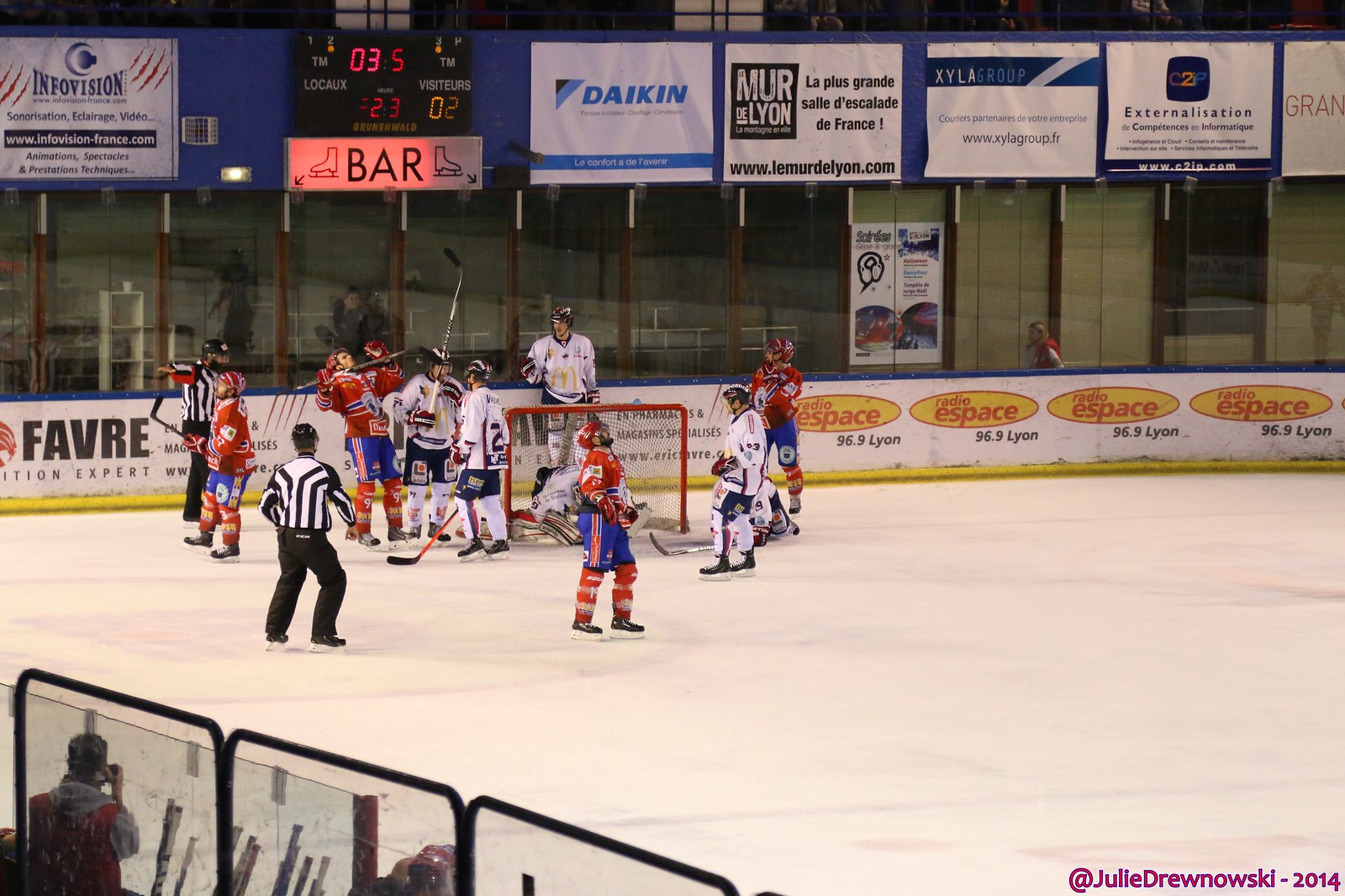This photograph captures an intense moment during a hockey game, shot from a vantage point overlooking the ice rink. On the ice, players from two teams are congregated around the goal. The team in red jerseys, blue pants, and red-and-white striped socks contrasts sharply with the team in white jerseys, black-and-white shorts, and white socks. Both team goalies can be seen near the net, accompanied by two referees in black-and-white vertically striped uniforms and black pants. The spectators are scattered in the stands located to the left, with protective glass barriers lining the rink's edge to guard against stray pucks. Dominating the background is a scoreboard displaying the score and time, marked with "Barr" underneath. Surrounding it are various advertisement banners in both French and English, including "InfoVision," "Dakin," "Murray and Lyon," "Xyla," "Xterminalitation," and "radio espace." The rink's boards are also adorned with ads, such as "Espace" in a yellow oval with red print, and "Favre" in bold black letters against a white background. The photograph is credited to Julie Junowski, 2014, as indicated by a watermark in the lower right.